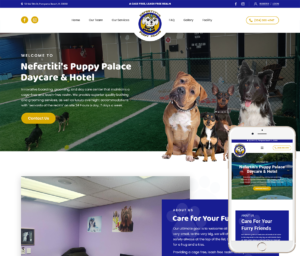The image appears to be of the website for Nefertiti's Puppy Palace Daycare and Hotel. The homepage features several sections, including Home, About Us, Pricing, FAQ, Gallery, and Facility, which are prominently mentioned. At the top of the homepage, there's a welcoming message: "Welcome to Nefertiti's Puppy Palace Daycare and Hotel." However, some smaller white text is unreadable due to its size and blurriness, likely providing additional information about the services offered.

Further down the page, there is a "Contact Us" button, along with icons linking to Facebook and Instagram, indicating the presence of social media channels. The website also showcases what appears to be an app, displayed through an image of an older white iPhone, though it's unclear whether it's an actual app or just the website accessed via an iPhone.

An incomplete piece of text reads "Care for your F.U.," which is likely intended to say "Care for your furry friends." Additionally, there is another image partially visible, and the website URL www.nefertiti.com can be seen at the bottom.

In summary, the image is a snapshot of Nefertiti's Puppy Palace Daycare and Hotel website, offering a range of services and accessible through social media and potentially a mobile app.